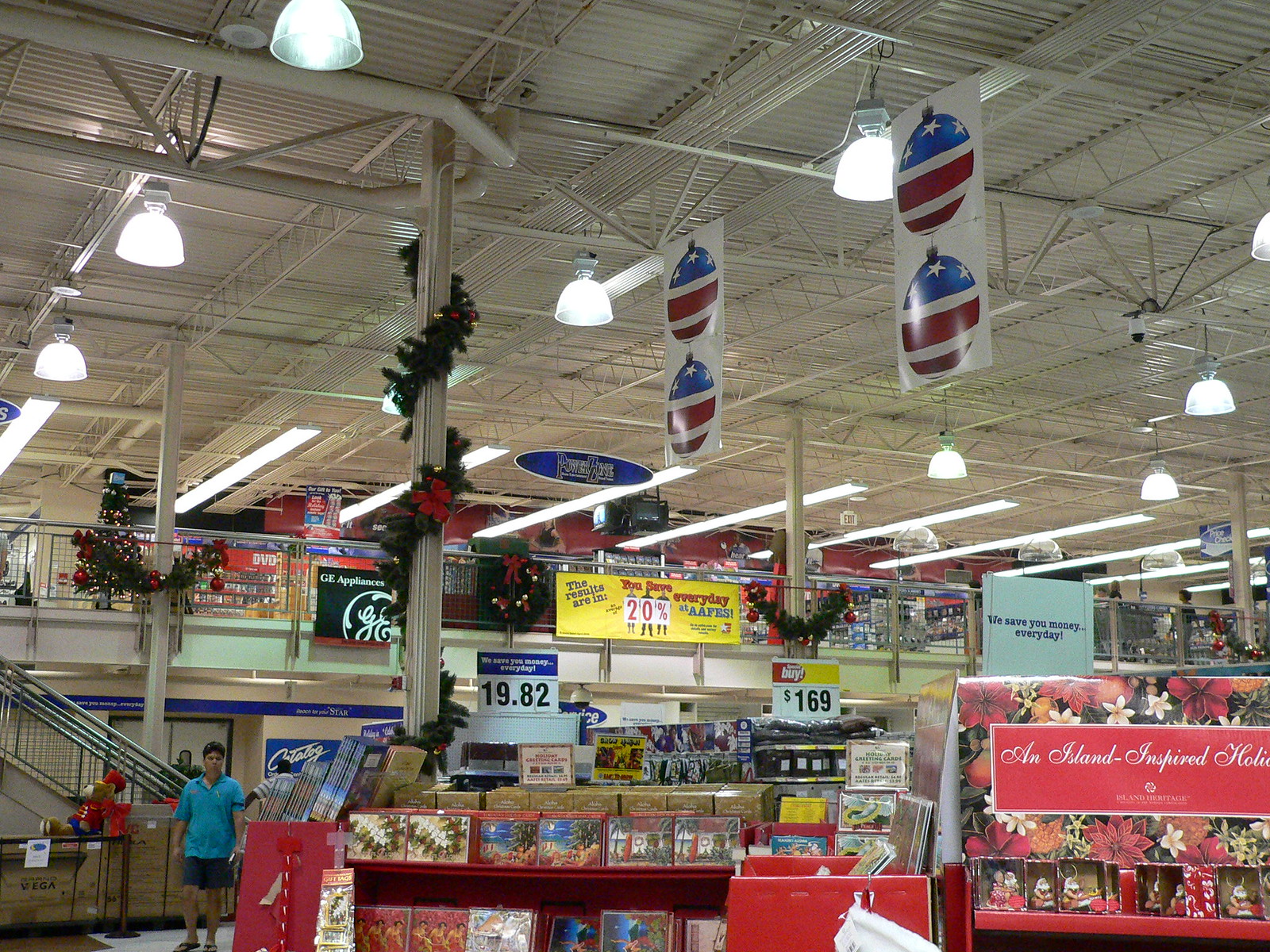The image captures the bustling interior of a supermarket, where multiple aisles are lined with a wide array of products neatly arranged on shelves. Festive cheer is evident as Christmas items such as cards and tree ornaments prominently feature. Brightly colored lighting hangs from the open ceiling, casting a warm glow over the scene. The photograph is awash with holiday hues, particularly reds and greens, enhancing the festive atmosphere. Shoppers meander through the aisles, absorbed in their tasks. In the background, a man in a blue shirt and gray shorts can be seen, adding a touch of humanity to the vibrant setting.